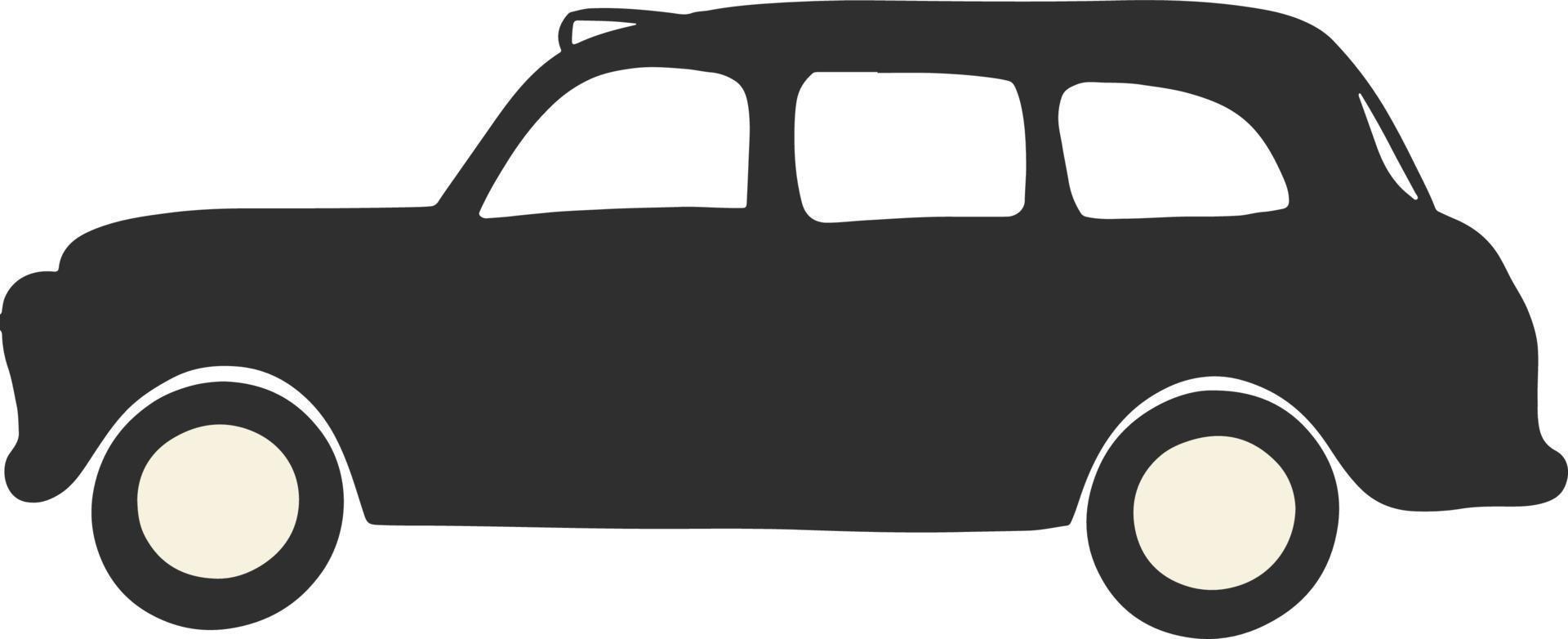The image depicts a simplistic, computer-generated silhouette of a notoriously rounded, vintage 1950s station wagon-like automobile. The car is entirely black, drawn in black ink, with no rendered details or markings, giving it a minimalist aesthetic. Noticeably bereft of sharp angles, the body of the car is strikingly smooth with rounded edges that characterize its old-fashioned design. The car features three distinctive windows along its side: a front oblong window, a square middle window, and a rear window shaped like half an eyeglass lens. The silhouette includes black tires with off-white rims, floating slightly disconnected from the car, and hints of a roof rack. The roof extends from a long hood, curving gently downward to where a trunk would be found on non-station wagon vehicles. The entire composition is simple and devoid of complex details, emphasizing the car's vintage, flowing shape.